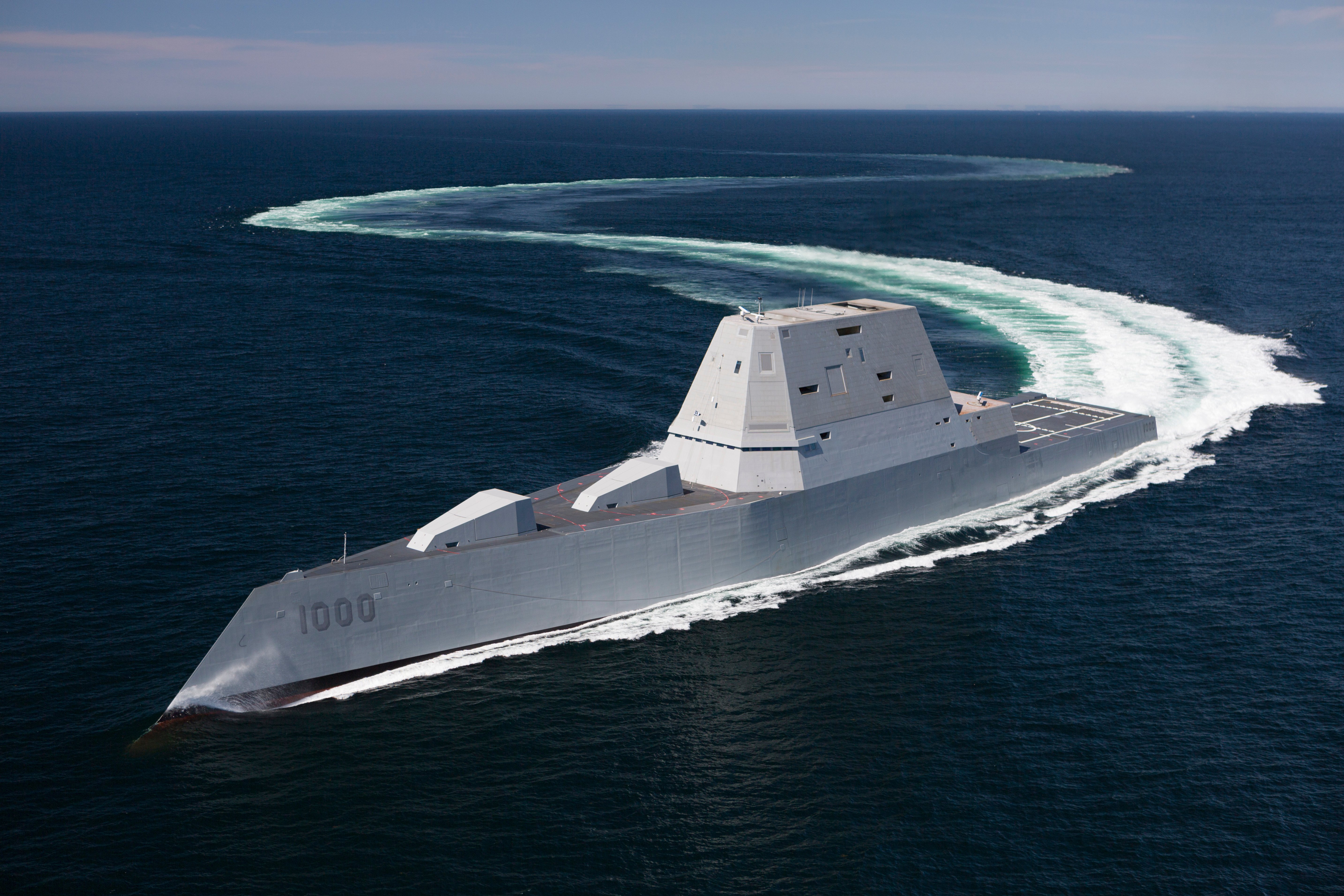The image showcases a vast, dark blue ocean under a sky with thin wispy white clouds and hints of pale blue and pink. Dominating the scene is a long, sleek, silver-white ship with a futuristic and military design. The ship's front curves sharply to a missile-like point, displaying the numbers "1000" prominently. At the center of the ship, there's a tan, triangular-prism-shaped elevated platform, and a white dome that adds to its imposing, modern appearance. The vessel moves swiftly, leaving behind a distinctive, frothy wake that forms an S-shaped path through the water, emphasizing its rapid progression. No people are visible on this ship that appears armored and ready for serious endeavors, contrasting sharply with the serene yet vast ocean around it.